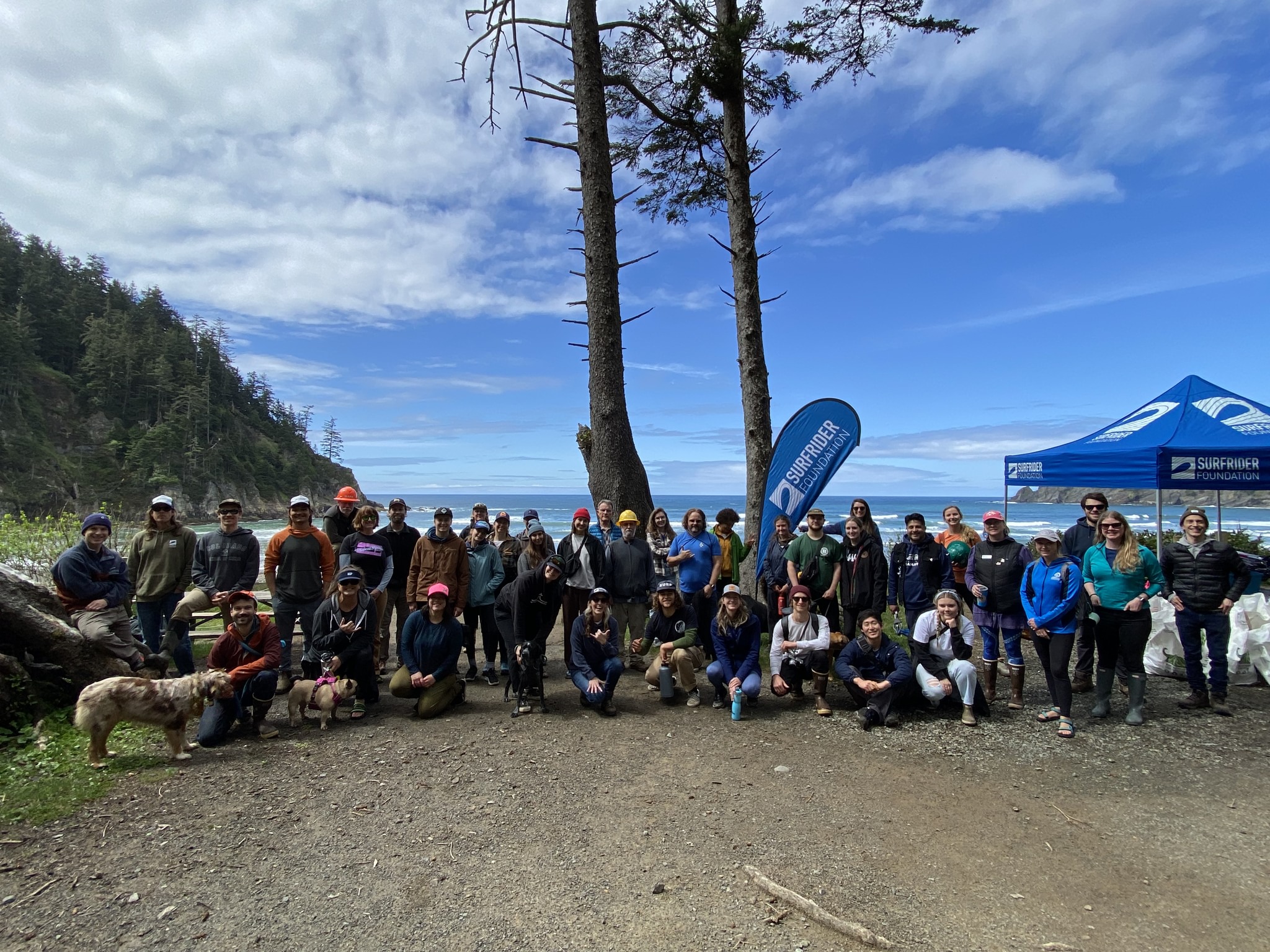A large group of 40 to 50 people is gathered outdoors in a dirt area, with a distant beach and ocean visible in the background. To the left, a tree-covered hill rises against a bright blue sky dotted with thin, wispy clouds. The group is casually dressed, with many wearing jeans, khakis, and long-sleeve shirts; some sport hats. In the front row, a few individuals kneel while the rest stand behind them. A blue tent bearing the label "Surf Rider" is set up to the right, along with what appears to be a paddleboard or oar cover also labeled "Surf Rider." In the bottom left corner, a man in a red hoodie kneels beside a brown and tan long-haired dog.